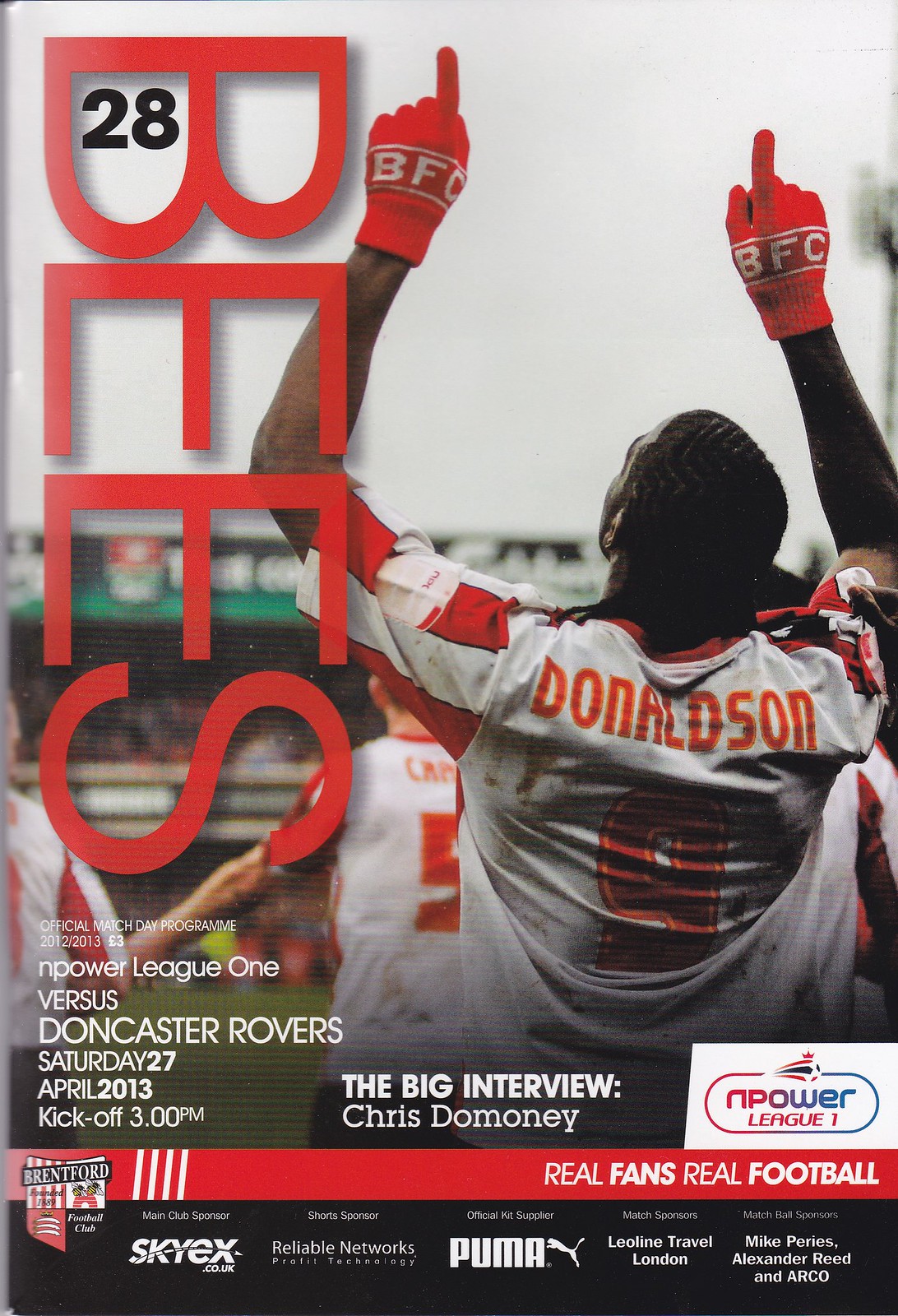The image is the cover of a scanned match day programme for an English football match, featuring Brentford Football Club versus Doncaster Rovers in the nPower League 1. Dominating the cover is a football player named Donaldson, wearing a white jersey with red stripes on the sleeves and an orange-bordered number 9 on the back. Donaldson is captured pointing both index fingers up to the sky, wearing red gloves with white "BFC" lettering, and has his hair styled in cornrows. The top left corner of the cover has the word "BEES" written vertically, with the number 28 inside the letter "B". Additional details on the cover include text highlighting "The Big Interview Chris Damone," the match date of Saturday, April 27, 2013, and the kickoff time at 3 p.m. Along the bottom of the programme, in a black bar, are various sponsor logos including SkyX.co.uk, Reliable Networks, Profit Technology, Puma, Leeline Travel London, Mike Aries, Alexander Reed, and Arco. The cover emphasizes the theme of "Real Fans, Real Football."